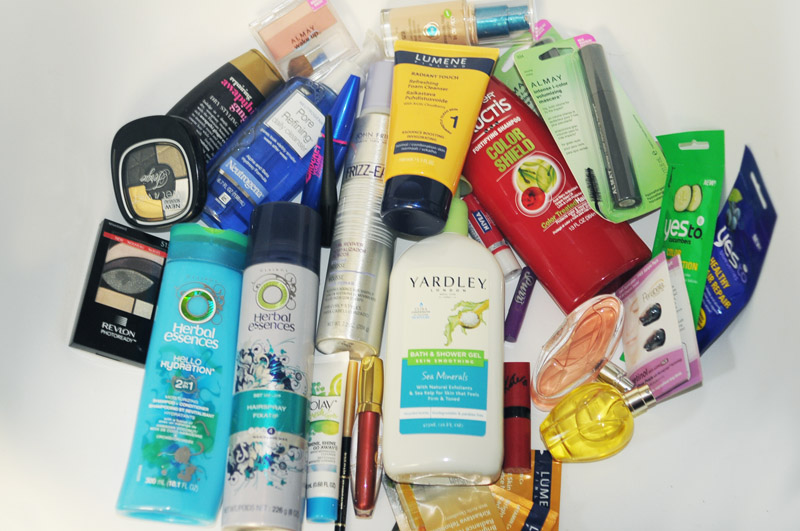The image features an assortment of hygiene products piled together against a white background. Prominently displayed are items from various popular brands such as Herbal Essences, Yardley, Lumine, and Almay. The collection includes a variety of containers and packaging types, illustrating the diversity of the products. There are plastic bottles with pumps, squeezable tubes without pumps, clear glass bottles, and even small plastic pods. The color palette is equally varied, with packaging in green, blue, pink, and transparent options. Among the products are shampoos, soaps, hair treatments, deodorants, and possibly perfumes or colognes, showcasing a comprehensive range of personal care items designed to cater to different hygiene needs.